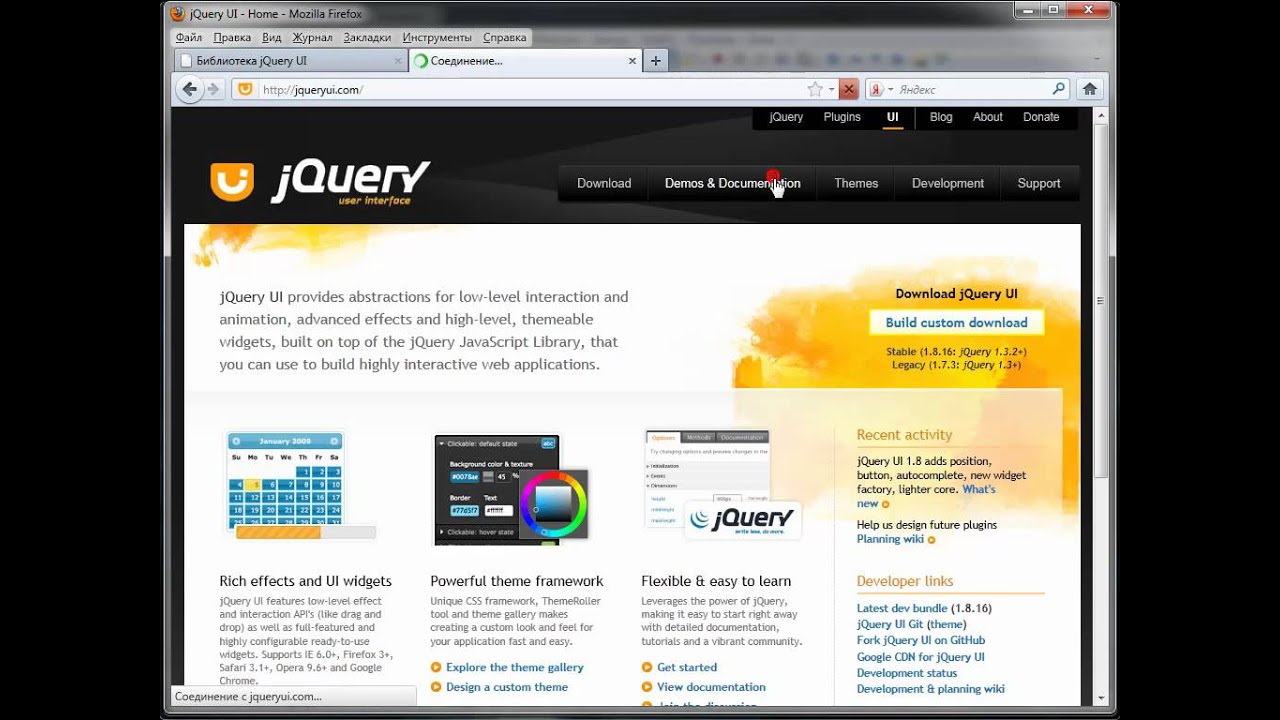The image depicts a user interacting with the jQuery UI website on Mozilla Firefox, accessible at http://jqueryui.com. The browser interface shows multiple groups of tabs, some containing Cyrillic characters. The webpage is navigated to the 'UI' section, indicated by a yellow underline beneath the 'UI' link in the top right-hand corner of the site menu, which includes links labeled 'jQuery', 'Plugins', 'UI', 'Blog', 'About', and 'Donate'.

Centered on the page is the jQuery UI logo, resembling a figure with legs together and raised, suggesting either a playful character or the letter 'J'. Below the logo, it says "jQuery User Interface". The page features buttons titled 'Download', 'Demos & Documentation', 'Themes', 'Development', and 'Support'. The user's cursor, marked by a red dot, hovers over 'Demos & Documentation'.

The central content area describes that "jQuery UI provides abstractions for low-level interaction and animation, advanced effects, and high-level, themeable widgets built on top of the jQuery JavaScript library, enabling the construction of highly interactive web applications." This text is set against a white background with artistic, ink cloud-like yellow and orange designs.

On the right-hand side of the page is a section focused on downloading jQuery UI, offering options such as 'Build Custom Download', 'Stable 1.8.16 (jQuery 1.3.2+)' and 'Legacy 1.7.3 (jQuery 1.3+)'. Below this, brief articles highlight the benefits of jQuery UI, such as "rich effects and UI widgets", "powerful theme and framework", and "flexible and easy to learn".

Finally, the right sidebar features two yellow-typed header sections titled 'Recent Activity' and 'Developer Links'.